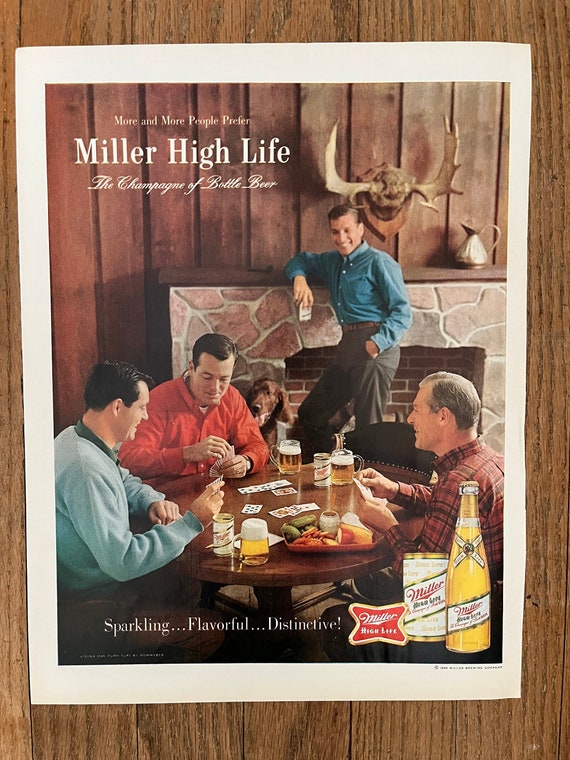This image captures a vintage Miller High Life beer advertisement from what appears to be the 1950s or 1960s, displayed on a piece of wood paneling. At the center of the ad, a scene showcases four men enjoying a game of cards in a rustic cabin setting. They gather around a round wooden table with mugs of beer, each with a foamy head, a couple of cans, and a plate of fruit. The man with black hair and a red shirt sits at the top center, drawing a card. To his left, another man with black hair wears a turquoise shirt, attentively watching the game. An older gentleman in a tan and brown plaid shirt completes the trio sitting at the table. Leaning against a stone and brick fireplace in the background is a man in a jade blue shirt, holding a can of Miller High Life, with his hand tucked into his pocket. Mounted antlers and a silver picture adorn the mantle above the fireplace, with an Irish Setter sitting near the man leaning against it. The top left of the poster features the Miller High Life slogan in white lettering, stating, "More and More People Prefer Miller High Life, the Champagne of Bottle Beer." The lower section of the ad, framed in a white border, highlights the words "Sparkling, Flavorful, Distinctive" in white letters against a black background, flanked by the red and gold Miller High Life logo and images of a Miller High Life bottle and can. The setting and attire suggest a convivial atmosphere reminiscent of mid-20th-century leisure.